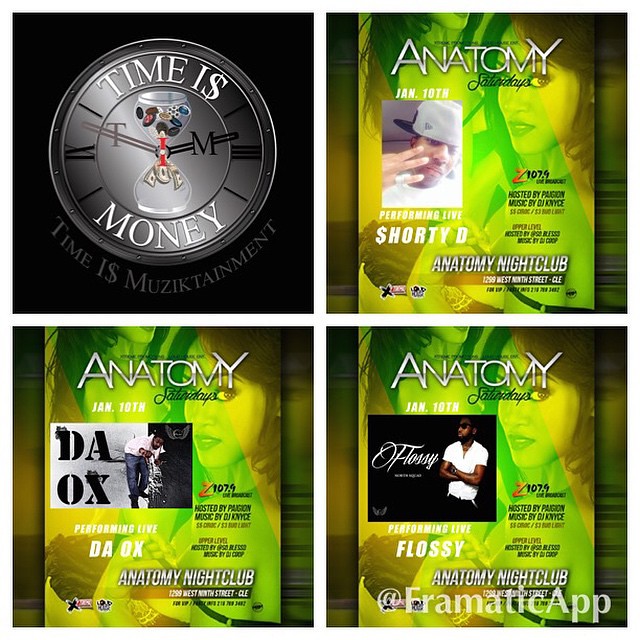The image is a collage divided into four sections, separated by thick white lines. In the upper left section, there's a clock with an hourglass at its center, symbolizing the concept of time turning into money as objects fall through the hourglass and transform into cash. The phrase "Time is Money" is prominently displayed on the clock, with the 'S' in 'is' represented as a dollar sign. Below the clock, in gray writing against a black background, is the modified phrase "Time is Musictainment," again using a dollar sign for the 'S' in 'is.'

The remaining three sections are green promotional posters for performances at the Anatomy Nightclub, located at 1299 West 9th Street, Cleveland. At the top, each poster mentions "Anatomy Saturdays" and the date "January 10th," with additional details including "Z107.9 hosted by Pyagon" and "Music by JD Nice." Each poster also features a background image of a woman looking toward the viewer.

- The upper right poster showcases Shorty D performing live.
- The bottom left poster features Da Ox, depicted in a white coat and blue jeans.
- The bottom right poster highlights Flossie, displayed with his arms folded and wearing a white shirt.